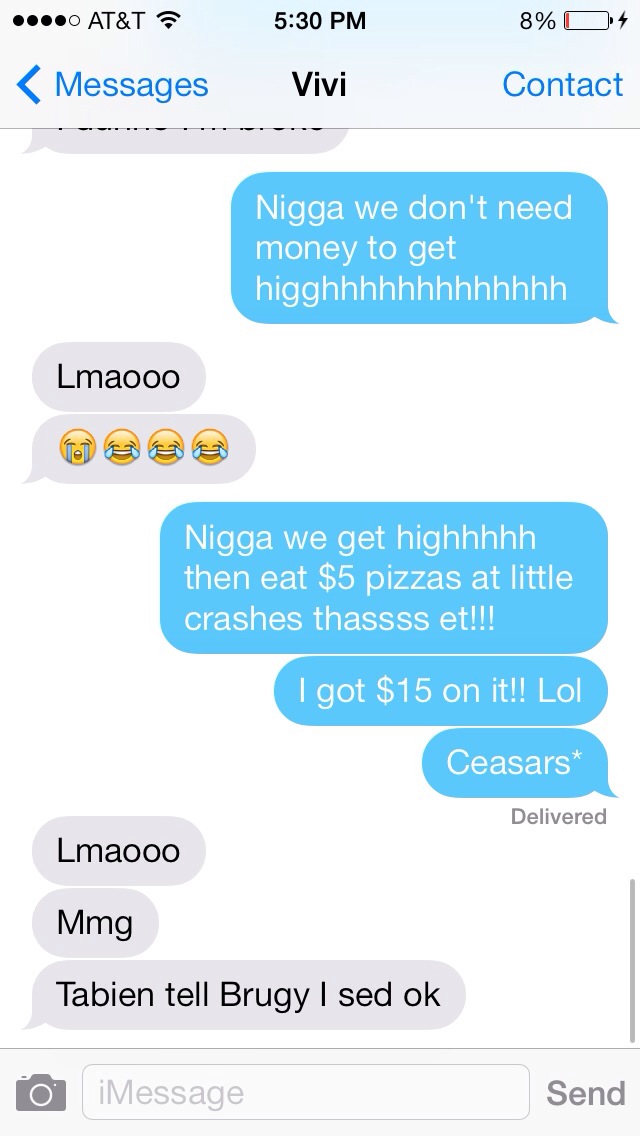This image is a screenshot of a smartphone displaying a text conversation. The phone belongs to an AT&T user with only 8% battery life remaining, and the time is 5:30 p.m. The screen shows a standard messaging interface with a white background, a light gray top section, and blue and gray text bubbles. At the top, there's a left-facing arrow labeled 'Messages' and a right-facing arrow labeled 'Contact,' with the contact name 'Vivi' in the center.

The conversation begins with a blue text bubble on the right, reading, "Nigga, we don't need money to get high," with the word "high" humorously extended as "H-I-G-G-H-H-H-H-H-H." The response from the other contact, in gray on the left, is "LMAO," followed by several crying and laughing emojis. Another blue bubble on the right continues, "Nigga, we get high, then eat $5 pizzas at Little Crash's. That's eat. I got $15 on it. LOL. Caesars," correcting the restaurant's name with an asterisk. The final gray bubble on the left responds with, "LMAO, MMG. Tambien, tell Broogie I said okay," with "said" misspelled as "S-E-D."

Below the conversation are the input text field and a 'Send' button on the right. Additionally, a small camera icon is located to the left of the input field, indicating an option to attach images. The entire chat showcases a casual and humorous exchange between friends planning a fun time.